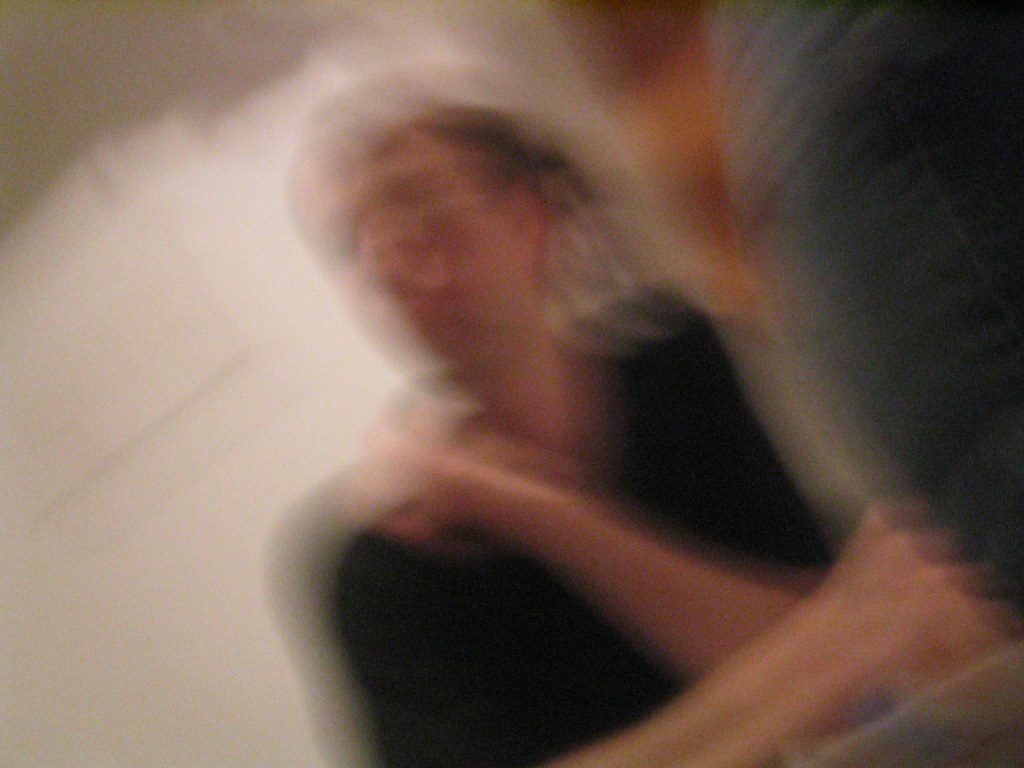A very blurred, horizontal image taken indoors captures a young white man in his early 20s, sitting at a table. The photo, shot from a very low angle almost at the surface of the table, shows the man slightly tilted in the frame. He has short brown hair and wears glasses along with a black collared shirt. His left arm is bent and raised across his chest, with his hand touching his right shoulder, while his right arm rests on the table in front of him. He is looking to his right (the left side of the image), seemingly distracted by something off-camera. The backdrop is a white color, and a spotlight appears to be shining on him. In the indistinct foreground, there is another figure or object near the lower right, almost out of focus and difficult to distinguish.